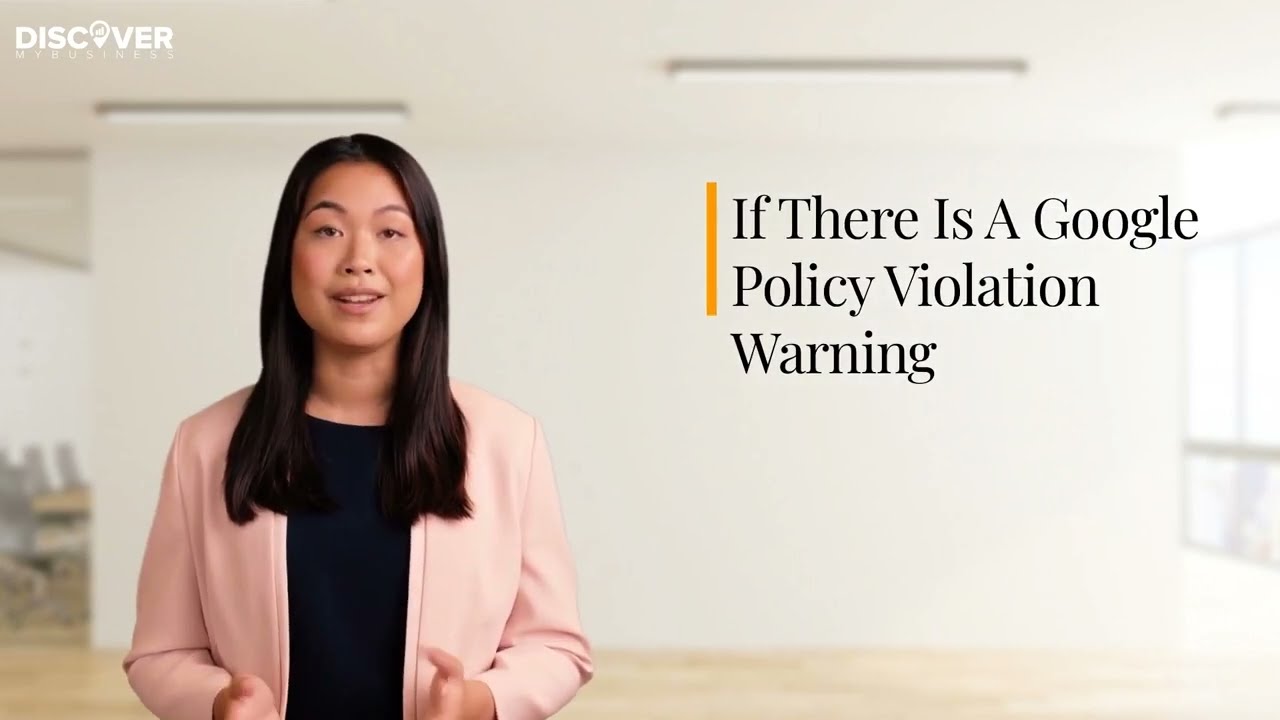An image captures a single Asian woman with long black hair, dressed in a peach-colored jacket over a black shirt, standing on the left side. Her hands are held up and forward as if she were holding something, and she appears to be in the midst of speaking or about to speak, with a slight smile on her face. In the top left corner of the image, there is a Discover logo with text related to "My Business." To the right of the woman, there's a Google policy violation warning in black text accompanied by a small yellow bar next to it. She stands in front of a spacious room with white walls and large windows that allow ample light to flood in, illuminating the wooden floor that has a light tan color. The backdrop behind her appears red with a large cinnamon background motif.